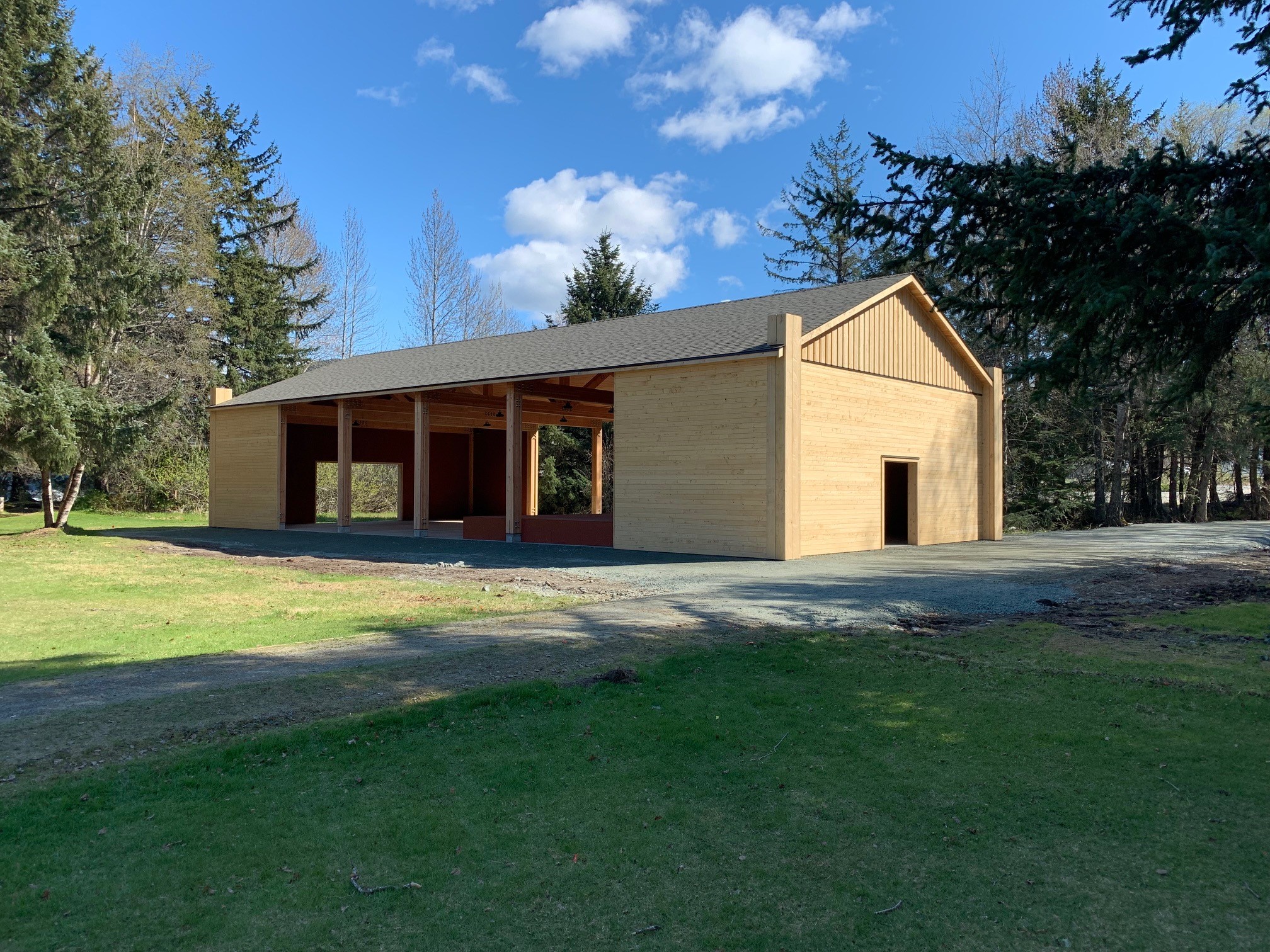A private driveway leads to a picturesque scene featuring a nearly-complete structure that resembles either a barn or a large shelter, set amid a lush, green landscape. On both sides of the driveway, evergreen trees such as Douglas firs frame the image. The main structure, centrally situated, is constructed from light tan wood and boasts a pointed, dark gray roof. The building, which could potentially serve as a barn, horse shed, or even a gathering place, has four open bays and small doors on both short ends, revealing an unfinished or open interior designed for easy access. While surrounded by meticulously maintained green grass with patches of brown, the structure is complemented by a light gray concrete path. A vivid blue sky with light, scattered clouds forms the serene backdrop, enhancing the rustic and tranquil ambiance of this secluded retreat.